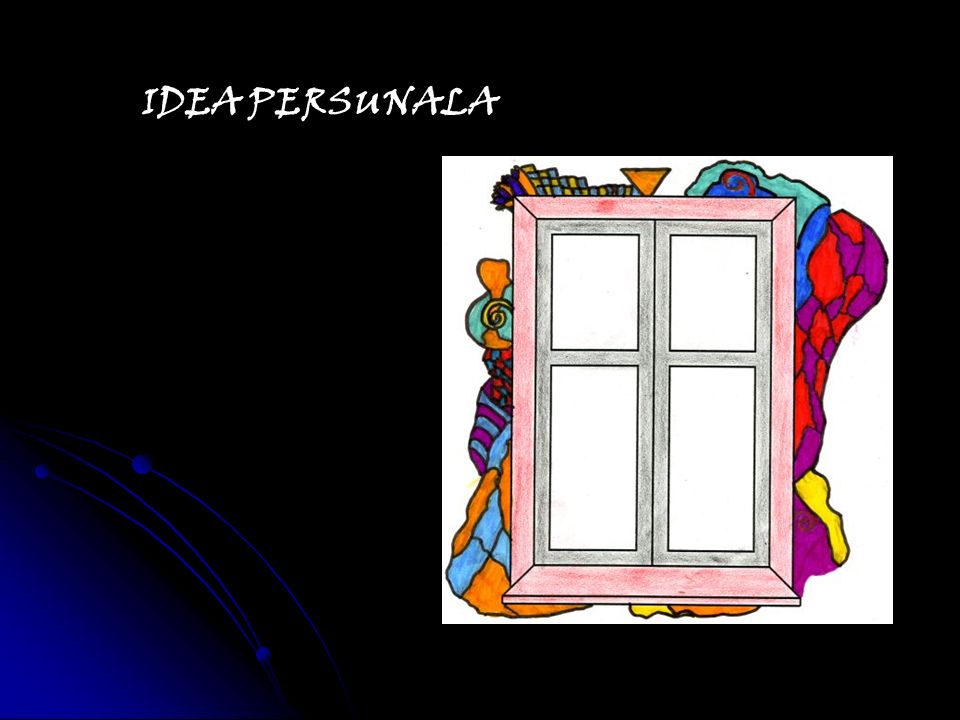The image features a predominantly black backdrop with a subtle purple tint and deep royal blue lighting in the lower left corner, evoking the appearance of a solar system with planets circumnavigating a larger celestial body. In striking white, bold, stylized text, "Idea Personala" is prominently displayed in the upper left corner. On the right side of the image lies a rectangular white box containing a hand-drawn window. This window has distinctive red frame and black grid lines, dividing it into four individual panes—two rectangular ones at the bottom and two square ones at the top. Surrounding the window are vivid psychedelic colors—yellow, red, purple, blue, orange—interspersed with various shapes, squares, and swirls, creating a dynamic and vibrant visual spectacle.